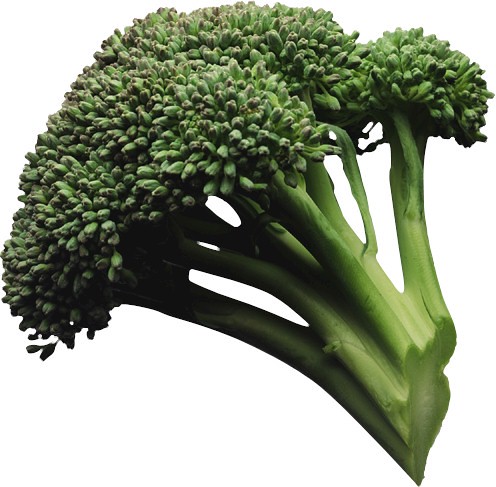This is a detailed close-up photograph of a fresh, robust head of broccoli with a clean, straight cut at the stem. The image showcases light green stalks and dark green florets against a white background, capturing the intricate tree-like structure. There are about nine to ten branching stems, ending in small, tightly packed green florets. The florets vary in color from bright green to a dark silvery-gray-green. You can see two distinct broccoli leaves growing off the main stalk, adding to the vibrant and hydrated appearance. The photograph is so close-up that individual sprouts and details like slight browning at the top and lighter shades in the cut stem are visible, providing a realistic and highly detailed view of the vegetable.